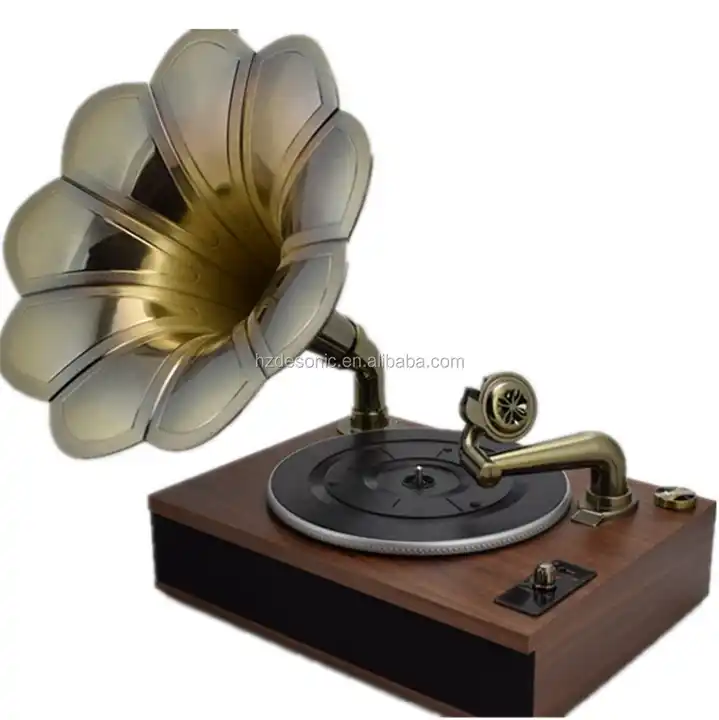This slightly out-of-focus image captures a beautifully crafted, antique-style record player. The record player sits against a plain white background, making it the central focus of the image. The device, which could be either a photograph or a computer rendering, features a wooden box base. At the center of the box is a black, round turntable with a silver spindle designed for mounting records. The turntable's needle is mounted on an ornate, gold-toned arm, styled in an antique fashion.

The box is adorned with a large, flower-shaped trumpet amplifier that extends proudly from its surface, adding an elegant touch. At the back-right corner of the box, there's a gleaming gold knob, while the front has two smaller round knobs—one on each side—situated on black rectangular bases. The box's front appears to be hollow or has a black panel, providing a subtle contrast to the rich wooden texture. The overall design and intricate details evoke a sense of nostalgia, capturing the charm of vintage audio equipment.